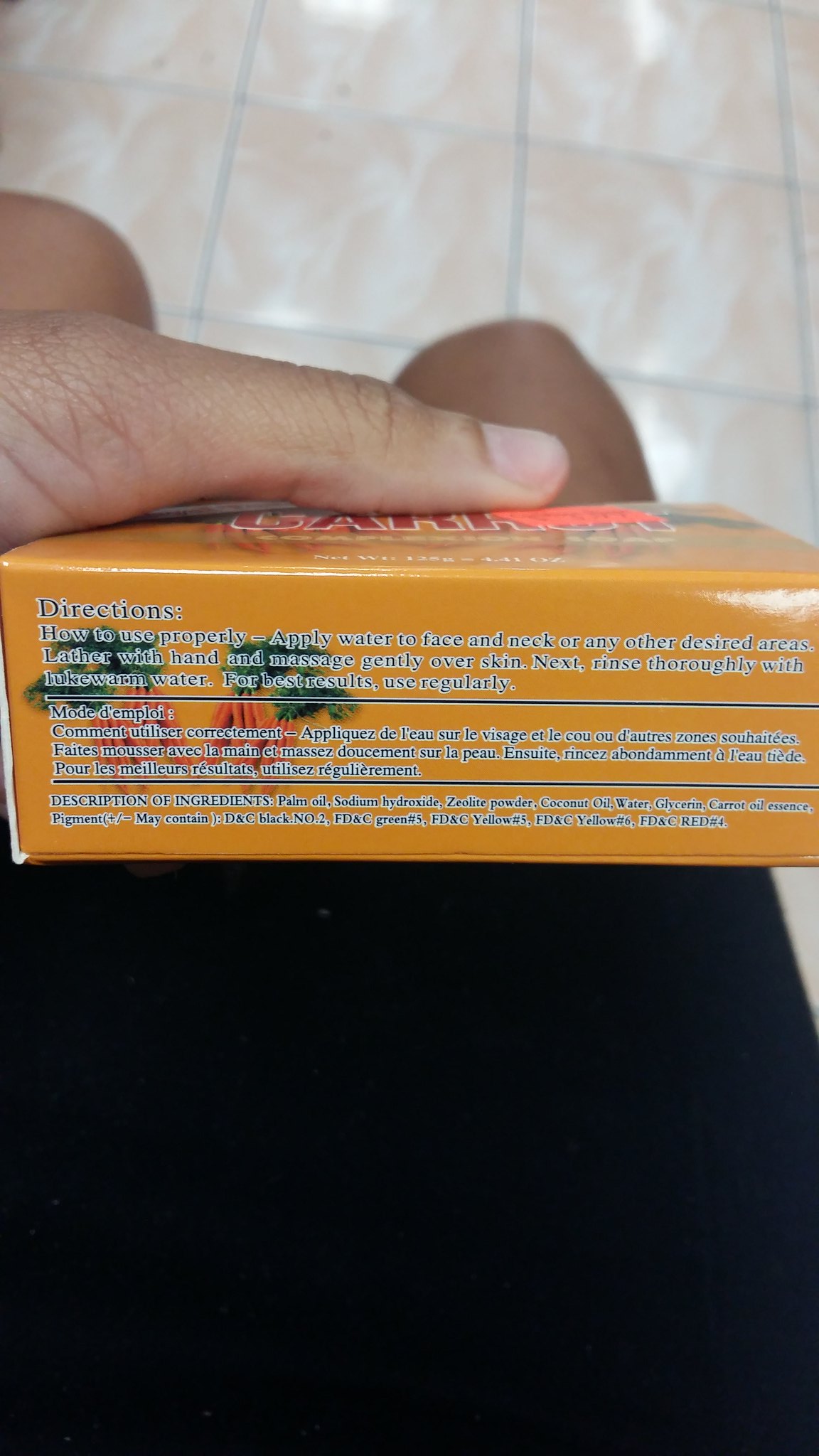A close-up photograph captures the bottom of a yellow-orange box being held by someone. The box features black text outlined in white, presenting the directions for use: "Apply water to face and neck or any other desired areas. Lather with hand and massage gently over skin. Next, rinse thoroughly with lukewarm water for best results. Use regularly." Below this text, a French translation of the directions is provided, followed by a description of the ingredients, including palm oil, sodium hydroxide, zeolite powder, coconut oil, water, glycerin, carrot oil, essence, pigment, and several color additives (DNC Black No. 2, FDNC Green No. 5, FDNC Yellow No. 5, FDNC Yellow No. 6, and FDNC Red No. 4).

On the left side of the box bottom under the directions, there are illustrations of four bunches of carrots with leafy tops. The top edge of the box is partially visible and appears to spell out "CARROT," though part of the word is obscured by an orange sticker. A forefinger is seen holding the box, with the person's knees visible below it. The lower portion of the image is predominantly black, while the upper part shows square linoleum tiles.